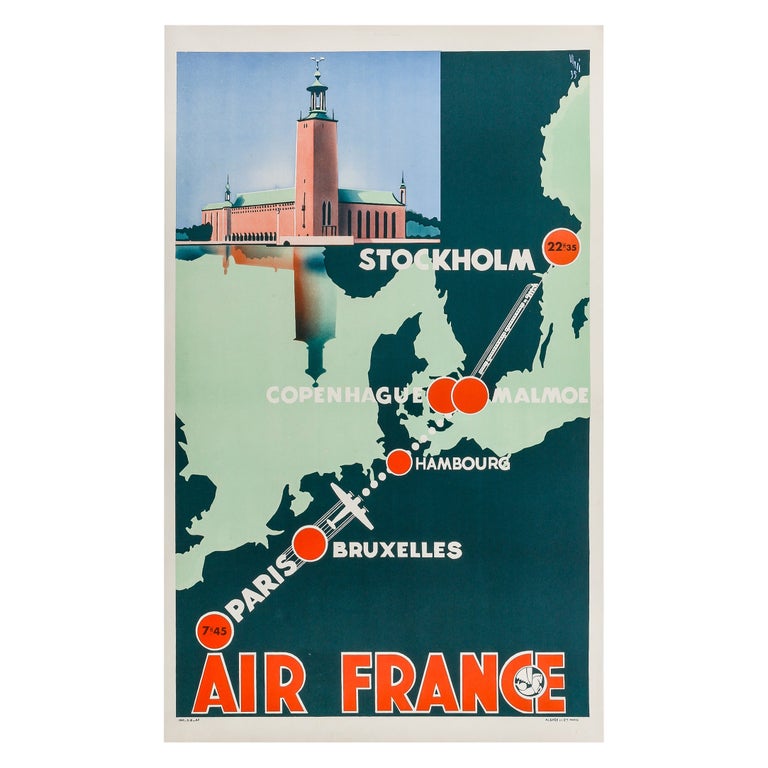This is a detailed Air France advertisement poster illustrating a flight route from Paris to Stockholm. The poster prominently features an outline of European countries in green, with the waters in lighter shades of green. Starting at Paris, marked with a red dot, the route continues through Brussels, Hamburg, Copenhagen, and Malmo, each designated by additional red dots, before reaching the final destination, Stockholm. At the bottom of the poster, the words "Air France" are boldly written in red. Additionally, specific flight times are indicated, with departure from Paris at 7:45 and arrival in Stockholm at 22:35. In the top left corner, there is a detailed drawing of a red-bricked airport with a high flight tower and glass windows at the top, resembling a lighthouse. At the bottom of this image, the word "Stockholm" is written in white. A small plane drawing traverses the route across the map, visually connecting the points of this international journey.